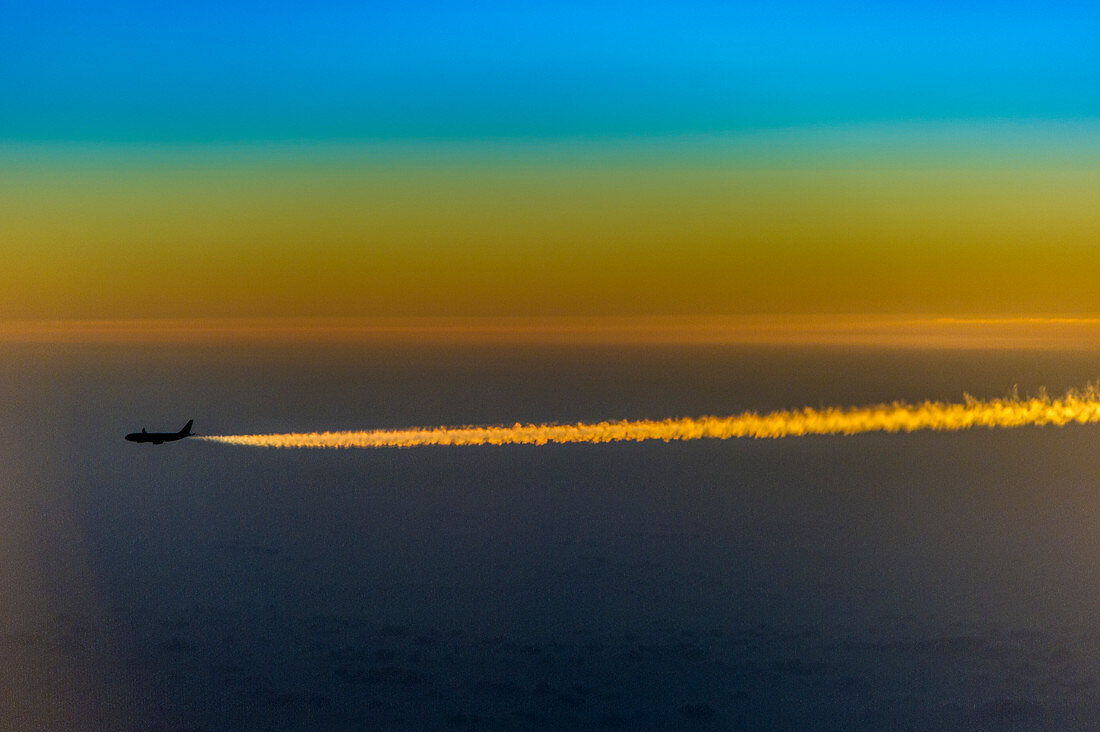This photograph, taken outdoors most likely at sunset, captures a dramatic and colorful sky with a silhouetted jet positioned towards the center left, streaking through the air. The jet leaves behind a striking jet stream painted in brilliant yellow hues, likely illuminated by the setting sun. The sky exhibits a mesmerizing gradient beginning with a deep blue at the top, transitioning through lighter blue shades into various shades of yellow as it approaches the horizon. Closer to the horizon, the color shifts into reddish tones, extending more prominently on the right than the left, before blending into a vivid yellow. Below the horizon, the hues change again to a greenish tint and finally into an aqua blue, tapering off into a truer blue, suggesting either water or land tinged with blue colors, possibly due to motion blur. The lower portion of the image shows a bluish area, hinting at a body of water or land. The sea or land beneath appears somewhat choppy or textured, further enhancing the complexity of this vibrant sunset scene.